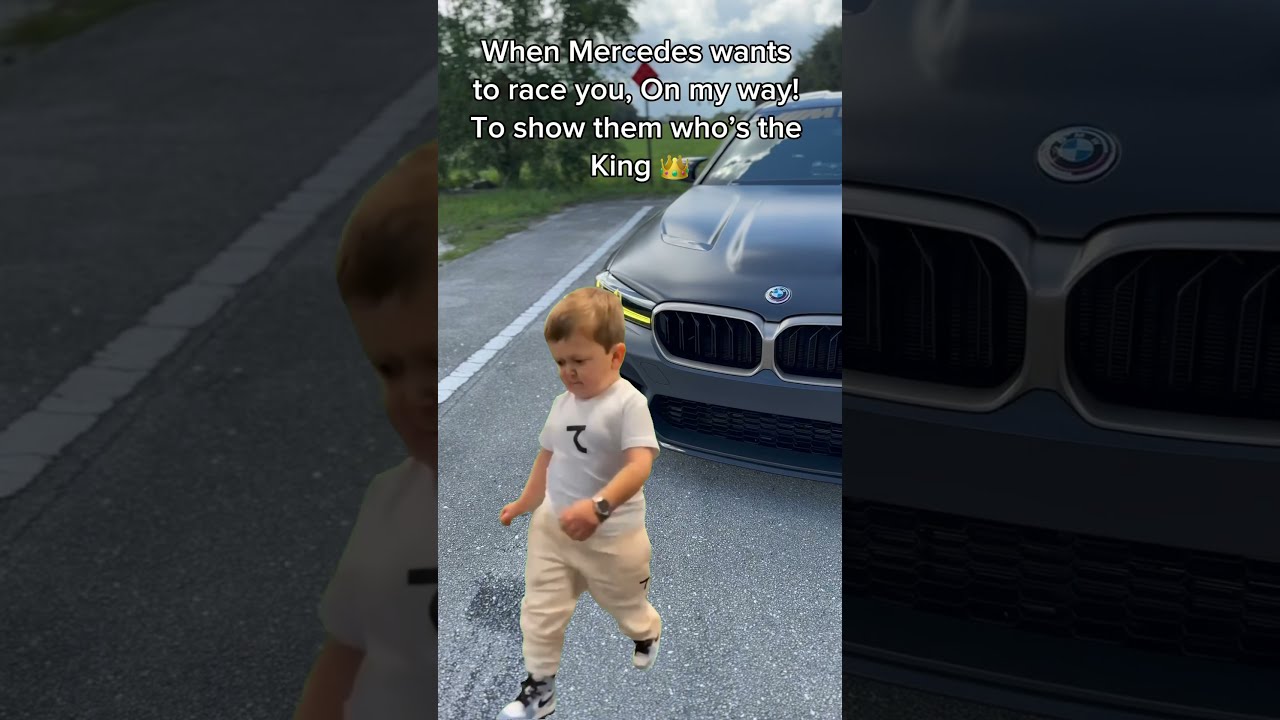In this screenshot from a video or reel, a young boy, probably around 8 years old, stands or runs in front of a parked, dark black or gray BMW on a paved road. The boy has light brown or goldish brown hair and is wearing a short-sleeved white t-shirt featuring a black character design, light tan or beige pants, and Nike shoes with a black swoosh logo. He also sports a watch on his left wrist. The image carries a humorous caption at the top in white text, saying, "When Mercedes wants to race you on my way to show them who's the king," accompanied by a gold crown emoji adorned with red and green gemstones. The backdrop includes a grassy field, a road sign, several green-leaved trees, and a blue sky dotted with clouds. The boy’s facial expression indicates he is not particularly happy, possibly grimacing or looking upset. This composition creates a playful scenario, comparing the boy's casual demeanor to the authoritative presence implied by the luxury car behind him.